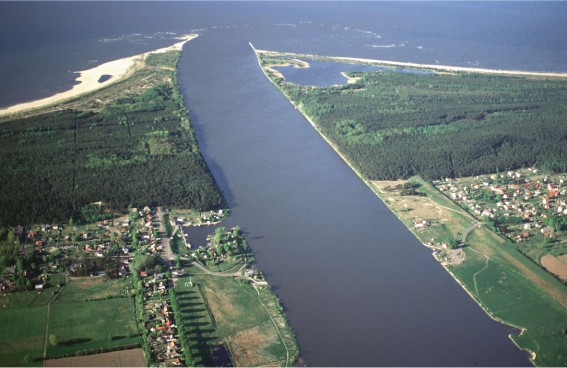A stunning aerial color photograph, likely captured by a drone, showcases a sprawling and diverse landscape. The image reveals a patchwork of clearly delineated parcels of land, which include what appears to be a mixture of farmland and forested areas. Interspersed throughout the landscape are several buildings, which may be homes or perhaps part of an industrial zone. Cutting through the center of the image is a narrow, dark waterway, its almost black waters creating a striking contrast against the vibrant greens and browns of the land. This waterway extends from the bottom of the image to the top, where it meets and feeds into a larger, expansive body of water. The top of the photograph is dominated by this larger lake or similar aquatic feature, emphasizing the blend of natural elements and human activity in this region.